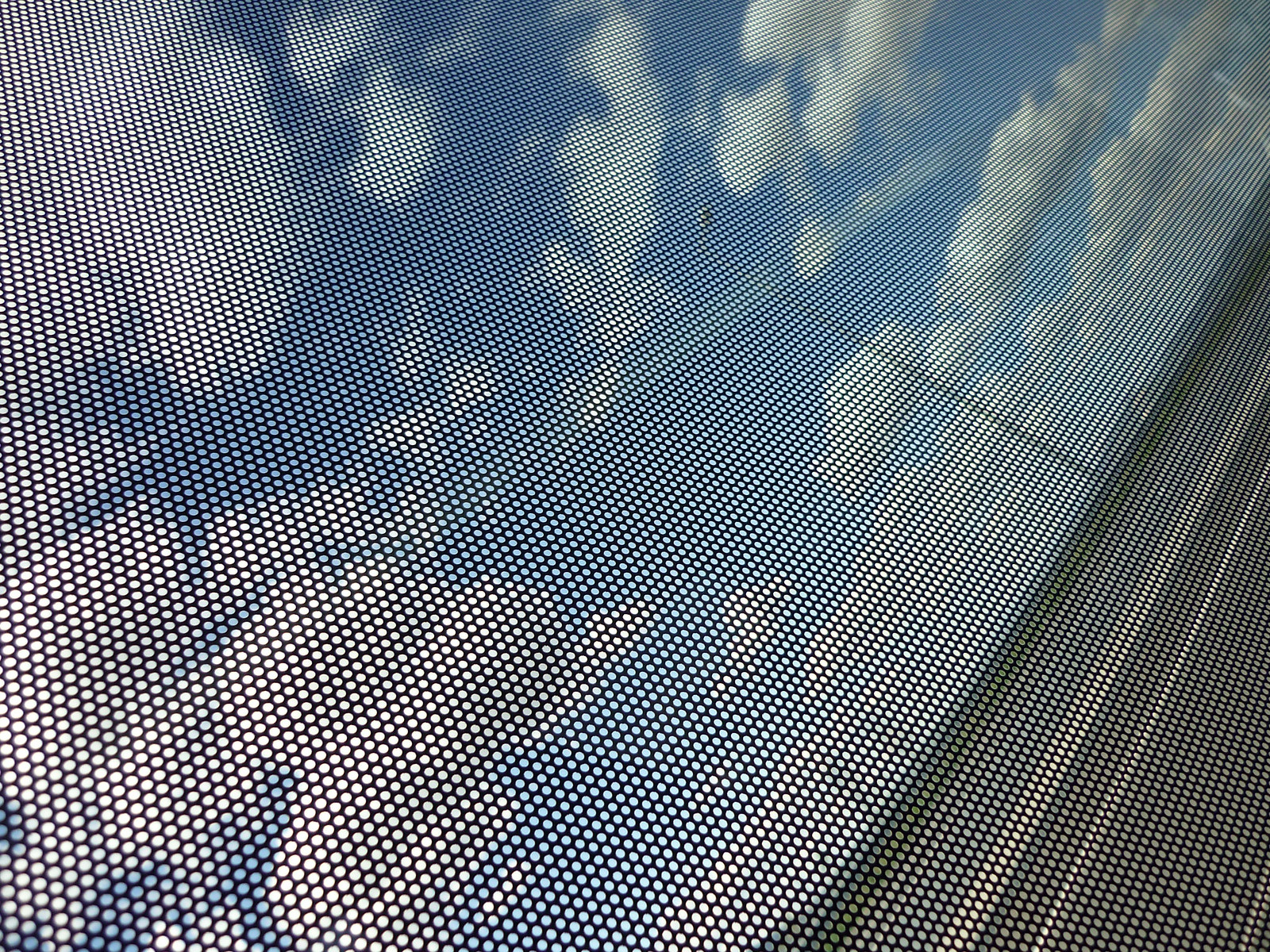This photograph, likely taken hastily or by accident from inside a public transportation bus, captures a tilted view of a highway scene at about a 45-degree angle to the left. The image is seen through a semi-transparent advertising sticker overlaying the bus window, allowing passengers inside to see out while obscuring the view from outside. The composition features a bright, partly cloudy blue sky dominating the left side while a road extends from the bottom right corner upwards, punctuated by a prominent street lamp centrally. Though the screen overlay affects visibility slightly, the vibrant day with its numerous fluffy clouds remains evident, imparting a surreal, almost staged beauty to the scene.